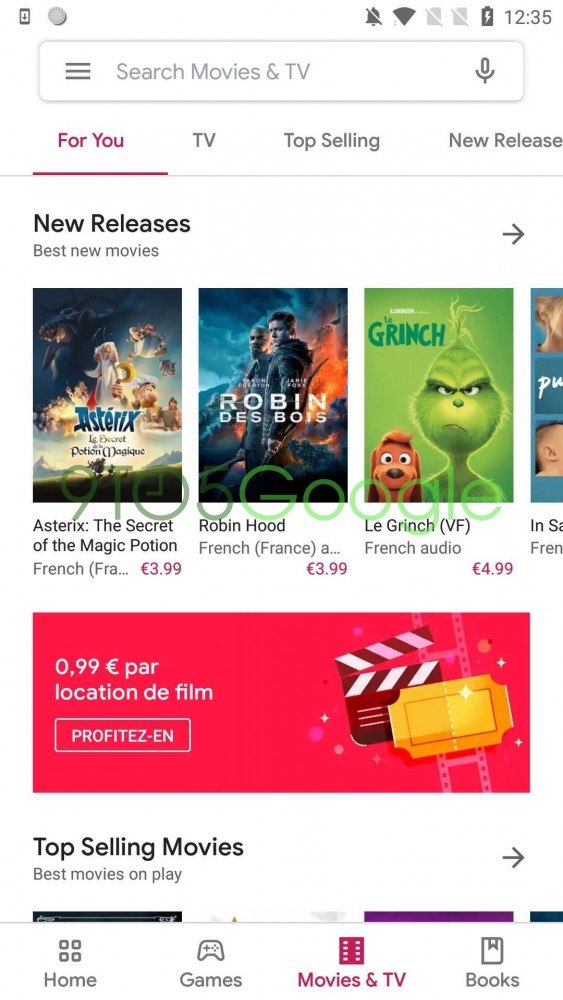The image captures the display of a webpage on a smartphone or tablet screen, detailed with various icons and navigation elements. 

On the top left, there is a phone logo accompanied by a down arrow. Next, a dark gray circle is present, followed by several notification icons. These include a bell icon with a line through it indicating muted notifications, a full WiFi symbol, and two light gray cell phone SD card icons each with a white line through them. There is also a battery icon showing a lightning bolt, likely indicating charging status. The time is displayed as 12:35, suggesting military time as there is no AM or PM indicator.

Below these icons, a search bar with a light gray border is positioned, containing an option to search for "movies and TV" in gray text along with a settings icon represented by three horizontal lines and a microphone icon for voice search.

The webpage features multiple tabs for navigation. The first tab, labeled "For You", is highlighted in hot pink with an underline, indicating it is currently selected. Other tabs titled "TV", "Top Selling", and "New Releases" are displayed in black.

In the content section, the "New Releases" headline, marked in bold black text, is followed by "Best New Movies" in gray. The section showcases various movie titles with associated prices. The first movie, "Asterix: The Secret of the Magic Potion", is labeled in French with the abbreviation (FRA) and priced at $3.99. "Robin Hood" follows, also in French, available for $3.99. The next movie, "The Grinch", listed as "La Grinch (VF)", is priced at $4.99, offering French audio.

A partially cut-off movie image on a blue background features Caucasian characters including a dirty blonde-haired woman and a buzz-cut man. Accompanying this is a hot pink rectangle stating "0,99 euro PAR location de film" (possibly a rental price). A golden clasp is depicted, along with a black and white striped movie action clapperboard, and a clickable white-bordered button labeled "Profitez-en" (Take advantage).

Below, in bold black text, "Top Selling Movies" is highlighted, followed by "Best Movies on Play" in regular black or gray text. Additionally, a black arrow is shown to the right-hand side.

At the bottom bezel of the screen, multiple clickable buttons for different sections of the app are visible. These include a "Home" button with a four-square icon, a "Games" button with a controller icon, a selected "Movies and TV" button in a purplish color with a building icon, and a "Books" button with a bookmark icon.